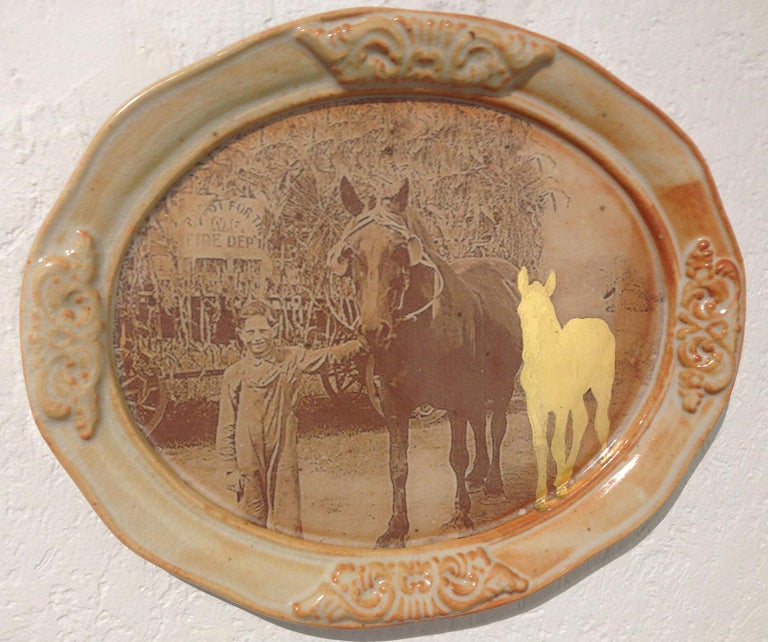This image depicts an oval ceramic serving platter, adorned with intricate raised details of abstract swirls and curves around its edges. The ceramic is primarily cream-colored, with a border accented by brown paint. The center of the platter features an old sepia-toned photograph that has been printed onto the ceramic surface. The vintage photo shows a young boy holding onto the halter of a horse standing beside him. Both the boy and the horse gaze towards the camera. In the upper left corner of the photograph, there is a sign that reads "fire department," and a wagon filled with tall corn stalks is visible. The background includes faint, possibly deteriorating, details that resemble trees. The overall appearance of the platter gives an impression of age and weathered beauty, contributing to its nostalgic charm.